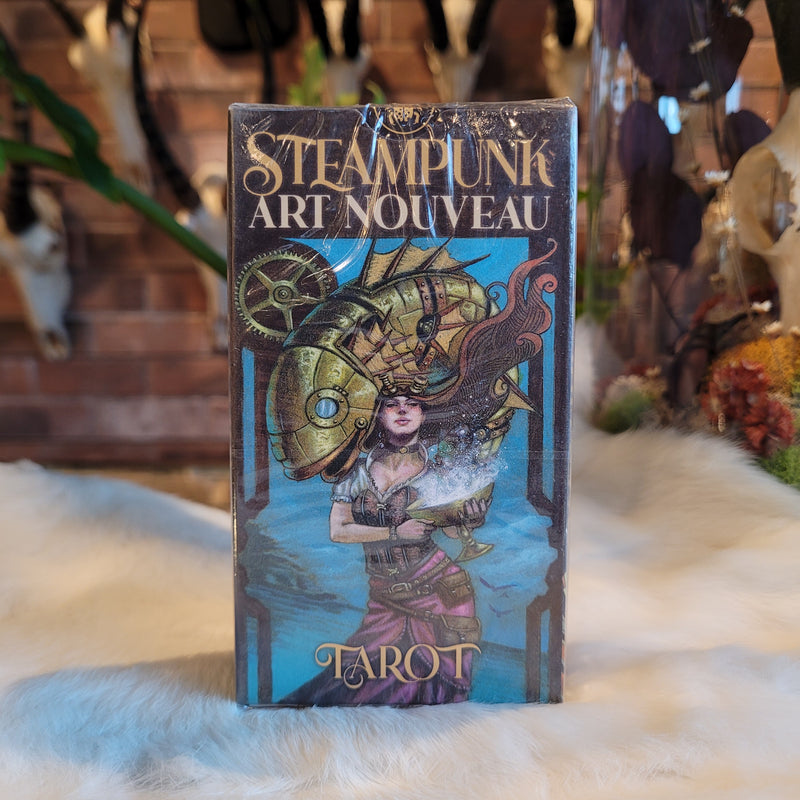The image is a high-quality, close-up photograph of a square package, approximately six inches by six inches, which is likely a set of tarot cards. The package, still wrapped in plastic, prominently features the title "Steampunk Art Nouveau" in gold and cream writing at the top on a brown background. Below this, against a blue backdrop, is an intricately detailed illustration central to the packaging's design.

The illustration depicts a Caucasian woman with long brown hair flowing to the right. She wears a large mechanical fish hat made of gold metal sheets with copper accents, including lips and a window for an eye. On her head also rest a pair of goggles. Her attire consists of a black choker, a brown bustier over a short-sleeved white blouse, and a pinkish-purple skirt with multiple brown belts, some featuring pouches. In her left hand, she holds a goblet emitting white, smoky potion-like wisps.

The word "Tarot" in gold print is displayed at the bottom of the package, solidifying its identity as a tarot card set. The package is situated on a white faux fur rug, which contrasts nicely with the background. The backdrop includes a brick wall with decorative elements such as antelope skulls and vases with flowers, suggesting a store or collectible display setting. The overall steampunk art style and vibrant colors of the package make it a visually striking product designed to capture attention.